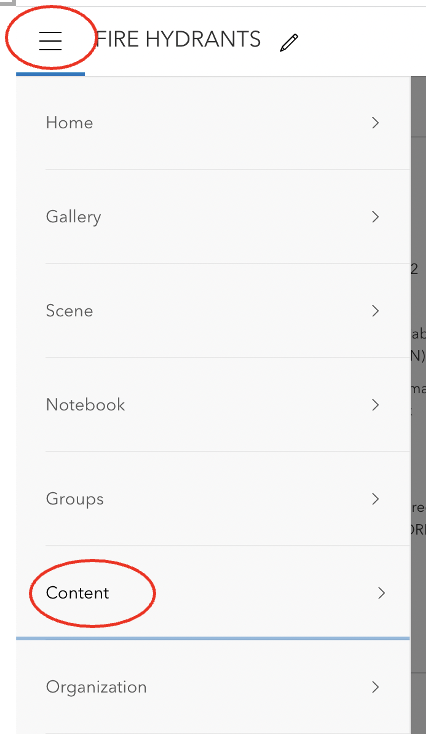The image features a white background with various graphical elements and text. At the top, a thick gray horizontal line spans the width of the image. In the top left corner, there is a slightly thicker gray square. Below this square, three gray lines are encircled in red. To the right of these lines, the words "fire hydrants" are written in gray font followed by a gray pencil icon.

Below this section, a thicker blue line runs horizontally. There’s a series of gray lines and shaded areas forming a table-like structure. A thicker gray line runs vertically down the right side to the bottom. Within this structure, the following elements are present:

- A lighter gray shaded area with horizontal text elements.
- The text "Home" followed by a right-facing gray arrow.
- Beneath, a gray line is followed by "Gallery" and another gray arrow.
- Below that, another gray line is followed by "Scene" and a green arrow.
- Continuing down, another gray line is followed by "Notebook" and a green arrow.
- Further down, another gray line is followed by "Groups" and a gray arrow.
- Another gray line is followed by a red circle encompassing the word "Content," with a gray arrow to its right.
- A blue line follows this, and below it, the word "Organization" is written, followed by another gray arrow.

The entire arrangement appears to depict a structured list or menu of some sort, with visual markers such as arrows and circles highlighting specific items.